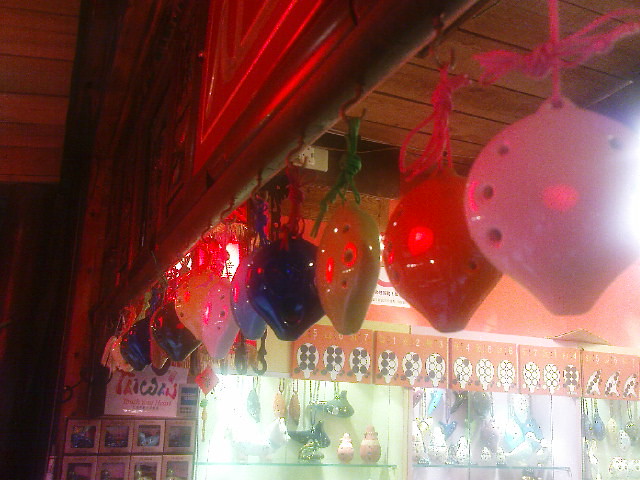This image captures a serene and inviting scene inside a charming Taiwanese shop, likely near its entrance. The ambiance is warm and laid-back, emphasized by an array of colorful, glass balloon-shaped ornaments hanging from a bamboo panel. These vibrant decorations, which come in heart shapes with three holes on each side, include various hues such as pink, red, yellow, blue, light blue, and white. Alongside these captivating ornaments, the shop features an assortment of pottery and decorative items, including a glass cat, pots, and teacups, highlighting a blend of traditional Chinese imagery. This tranquil setting, filled with artistic and cultural elements, invites a relaxed and enjoyable experience for visitors.